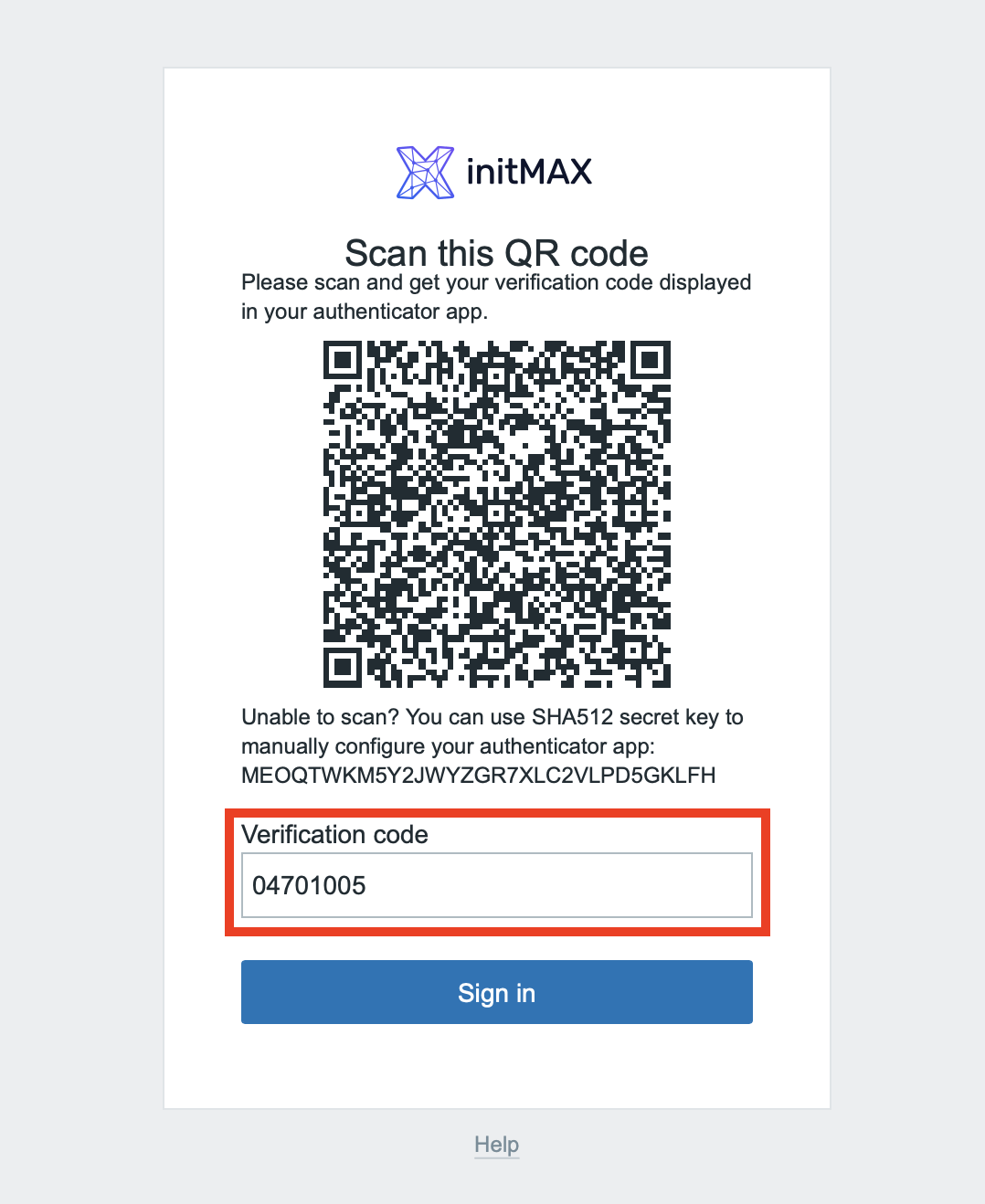The image features a gray background and prominently displays a large blue "X" with the text "MAX" (capitalized) underneath it. Below the "X," there is a prompt that reads, "Scan this QR code to get your verification code displayed in your authenticator app." Accompanying the QR code is a message that provides instructions for those unable to scan the code: "If you are unable to scan, you can use the SHA-512 secret key to manually configure your authenticator app." The secret key is given as "MEOQTWKM5Y2JWYZGR7XLC2BLPD5GKLFH."

To the right of these instructions, a red rectangle encloses the verification code "04701005." Below this section, there is a blue rectangle with white text that says "Sign In." At the bottom middle of the image, the word "Help" is written in blue.